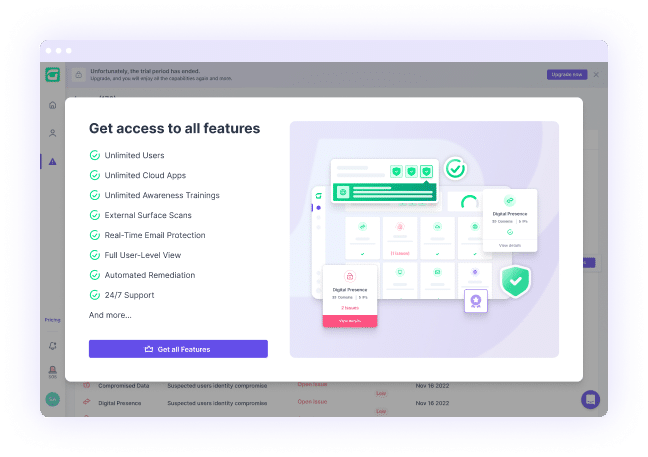This is a screenshot of a web page that has been mostly grayed out, highlighting a prominent, large white rectangular box that covers approximately 85% of the page. Within this white box, there is a well-organized layout featuring a column of text on the left and several images on the right.

Starting with the left column, at the top, it prominently displays the heading "Get Access to All Features" written in bold black text. Below this heading is a comprehensive list of features, each marked with a green circle containing a green check mark to its left. The features listed are as follows:
- Unlimited users
- Unlimited cloud apps
- Unlimited awareness trainings
- External surface scans
- Real-time email protection
- Full user-level view
- Automated remediation
- 24/7 support
- And more

Beneath this list, at the bottom of the left column, there is a horizontally oriented purple rectangle with a call-to-action button that says "Get All Features" written in white text.

To the right of this text column, there are several images showcasing different functionalities of the application. These images include square icons, check marks, and small purple ribbons, each representing a distinct feature or service offered by the site. The visuals provide a pictorial depiction of the site's services, complementing the detailed list on the left.